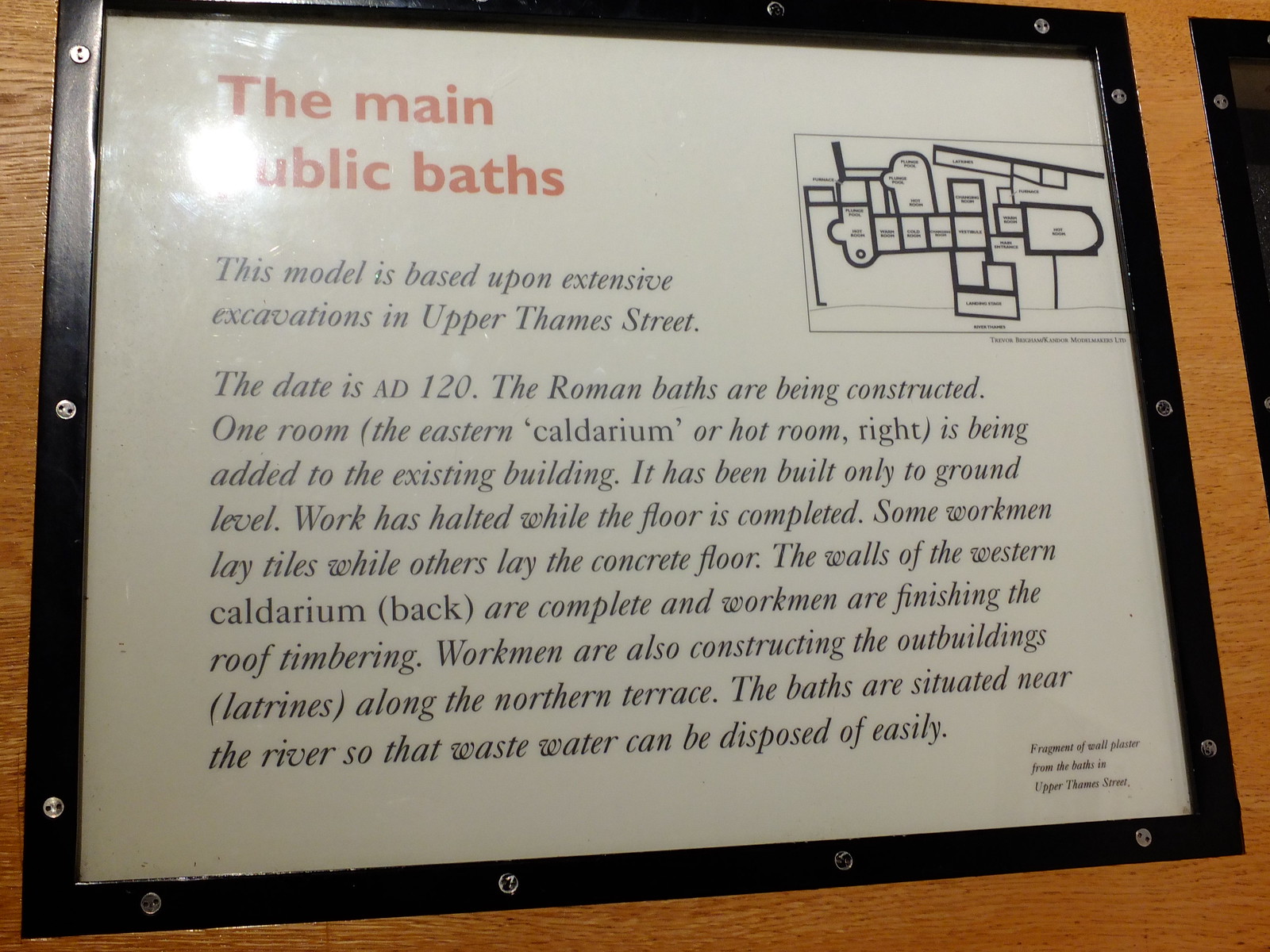The image captures an informational plaque titled "The Main Public Baths," mounted on a brownish wooden wall behind a black, square frame. The plaque features a predominantly white background with black text, while the title stands out in orange. Adjacent to the boldly labeled title, "The Main Public Baths," is a detailed diagram illustrating the layout of the Roman baths, consisting of various small squares, rectangles, and distinctive shapes that represent the different chambers and structures, including an upside-down can-like shape marking specific areas.

The text on the plaque provides a historical account based on excavations in Upper Thames Street, indicating that the Roman baths date back to A.D. 120. It describes the construction phases of the baths, highlighting the addition of the eastern caldarium (hot room) to the existing structure up to ground level, where work has paused for floor completion. Workmen are depicted laying tiles and concrete floors, constructing roof timbers on the western caldarium, and building outbuildings such as latrines along the northern terrace. The narrative concludes by noting the baths' strategic location near the river for efficient wastewater disposal. 

In the lower right corner of the plaque, a section with credits is visible, although the text is too small to read clearly. Reflecting light in the upper left-hand portion suggests the plaque is covered in protective plastic. Another similar but partially visible plaque is positioned to the right. This descriptive plaque likely belongs to an exhibition on Roman Britain, detailing the architectural and functional aspects of the ancient public baths.